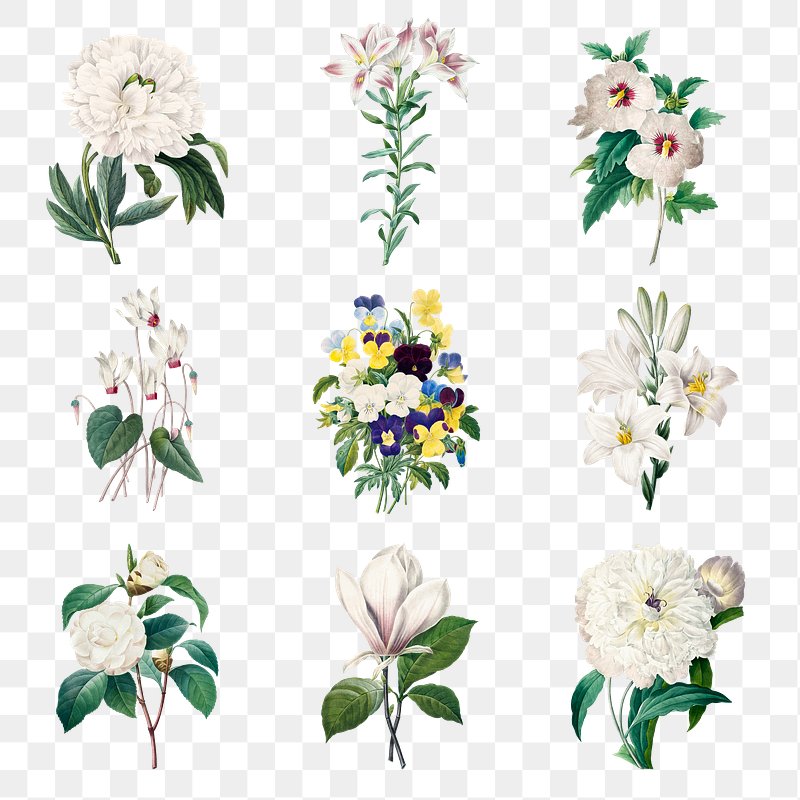This image presents a collection of floral clip art set against a classic gray and white checkerboard background. The arrangement consists of a grid with three flowers across and three down. Beginning from the top left, the first is a white chrysanthemum accented with green leaves. Adjacent to it is a pink and white lily with a long, leafy stem. The third in the row is a white flower featuring a yellow center and lush green foliage.

In the central row, the leftmost flower is another white bloom, this time with sizable leaves, followed by a vibrant assortment of small buttercup-like flowers in yellow, purple, white, and blue, all surrounded by green foliage. On the right, there is another white lily with subtle pink accents.

The bottom row begins with another white flower, possibly a type of chrysanthemum, to the left. In the middle is a white flower with green leaves, while the rightmost image features a peony with white petals and a hint of purple at its center. This diverse floral arrangement showcases a variety of blossoms, predominantly white, interspersed with colorful blooms, all vividly detailed against the distinctive checkerboard backdrop.